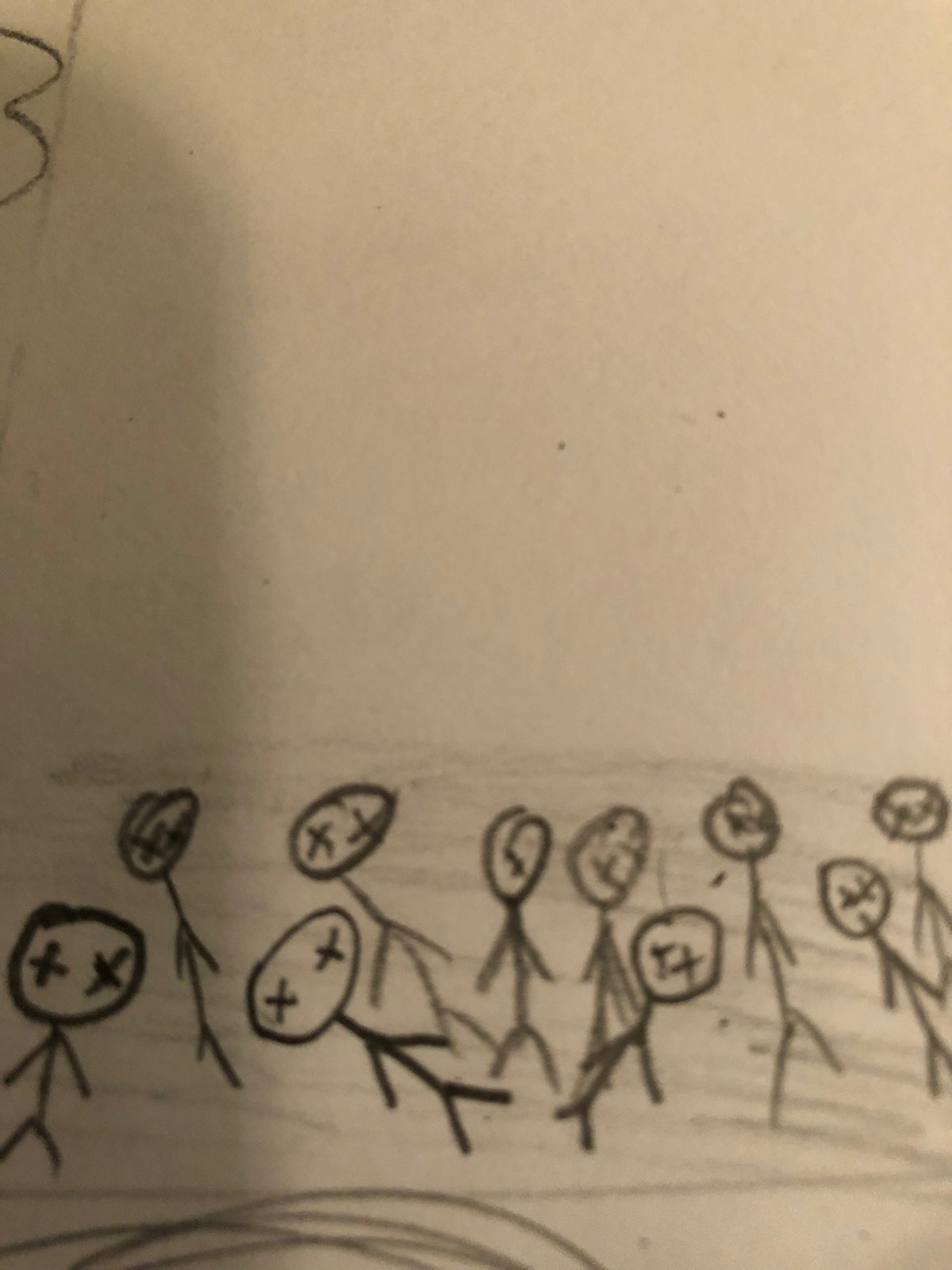The image features a childlike, morbid drawing on a sheet of tan-colored paper, likely done with a black crayon or a thick charcoal pencil. The paper has a slightly dirty appearance. The focal point of the drawing is a collection of 11 stick figures at the bottom, each with two stick arms, two stick legs, and round or oblong heads marked by X’s for eyes, giving them a lifeless appearance. Some of the figures are depicted walking, swaying, or laying on the ground, contributing to the eerie atmosphere. The ground itself is loosely shaded with darker scribbles towards the bottom, suggesting more detail that isn't fully clear. The top left corner of the image includes an indecipherable scribble, partially cut off, with shadows cast on the left side, adding to the drawing's overall somber tone. The composition is mainly negative space, with the morbid stick figures standing as the primary, unsettling focus.